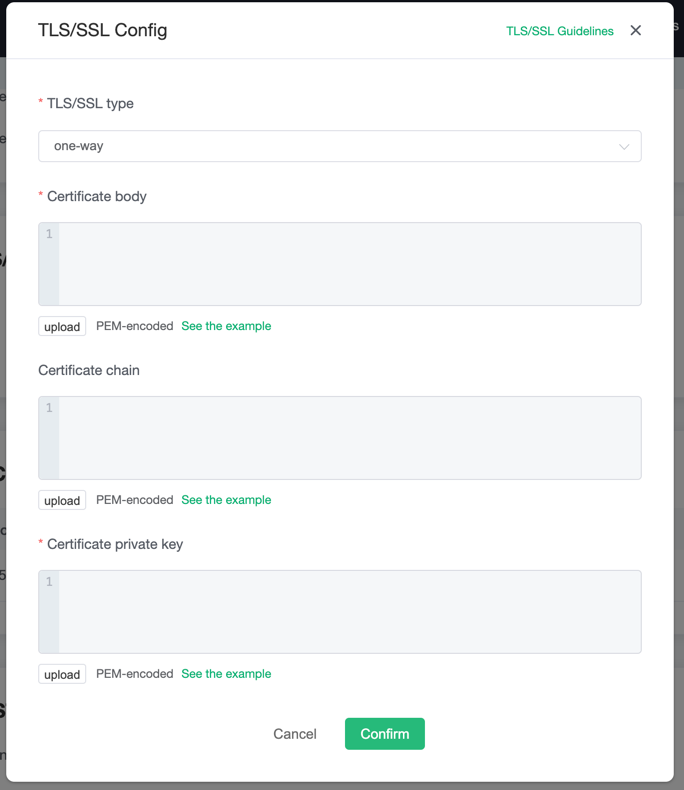The image depicts an online form related to TLS/SSL configuration, featuring a clean, minimalist design in white with black and green text. 

### Top Section:
- **Top Left Corner:** In bold, capital letters: "TLS/SSL." 
- **Right beside it:** The word "Config" where "Config" is capitalized.
- **Top Right Corner:** In green, uppercase letters: "TLS/SSL Guidelines" with a prominent black "X" icon next to it for closing the form.

### Form Fields:
1. **TLS/SSL Type:**
   - Marked with a red asterisk, indicating it is a required field.
   - A dropdown box with the option "One-way" selected.

2. **Certificate Body:**
   - Another red asterisk marks this as required.
   - A gray, shaded rectangle for users to input data.
   - Below it, in smaller text: "Upload PEM encoded. See the example."

3. **Certificate Chain:**
   - A gray rectangle similar to the previous field.
   - Information below: "Upload PEM encoded. See the example."

4. **Certificate Private Key:**
   - Marked with a red asterisk.
   - Another gray rectangle for input.
   - Small text below reads: "Upload PEM encoded. See the example."

### Bottom Section:
- **Cancel Button:** A standard cancel option.
- **Confirm Button:** A green box with white lettering reading "Confirm," indicating submission.

Overall, the form appears organized and user-friendly, guiding the user through necessary steps of TLS/SSL configuration.